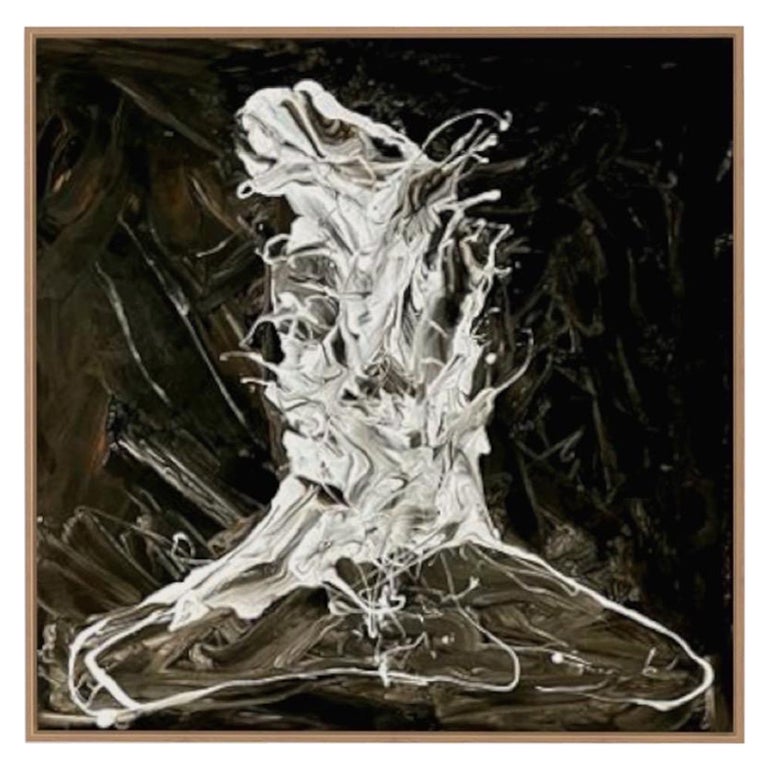The painting is a large, abstract work with a strikingly high-contrast palette primarily featuring black, dark brown, and white. The orientation is portrait, and the backdrop consists of various shades of dark brown and gray, creating a stark, somber atmosphere. Dominating the center is a vertically-oriented, milky white form that appears almost liquid-like, reminiscent of a watery, ivory-colored substance. This central element spreads out towards the bottom with long, stringy strands extending from its main body. The right side of the image is notably darker than the left, exhibiting more black and dark brown tones, while the left side shows some lighter brown accents. The painting is bordered in light brown and lacks any text or defining symbols, focusing purely on the abstract visual. Despite the poor quality of the image, its deliberate lack of clear representation and intricate interplay of contrasting shades emphasize its abstract style.